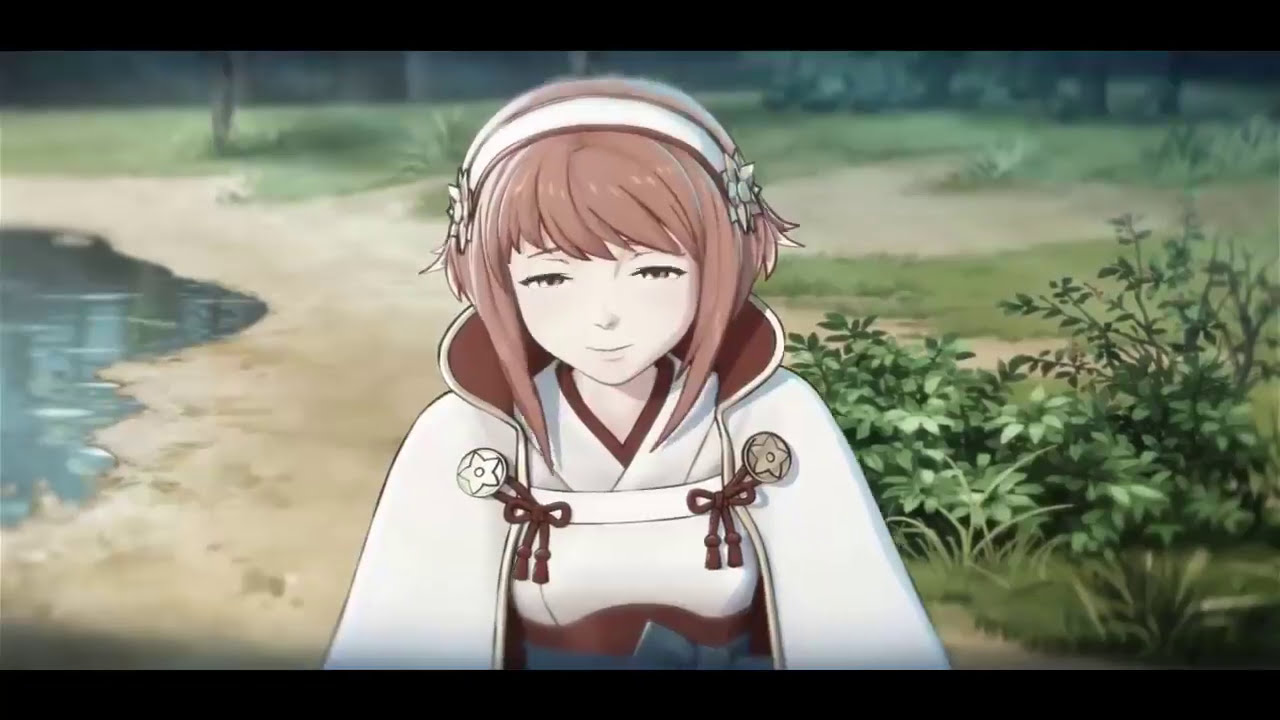The image appears to be a still shot from a Japanese or Korean anime, showcasing a female character who resembles a teenage girl. She is prominently placed in the center of a high-definition, widescreen frame with black borders on the top and bottom, giving it a cinematic aspect ratio. The girl has brown hair adorned with a white headband and is dressed in traditional East Asian attire that evokes historical Japanese or Korean fashion.

She wears a long, mostly white dress accented with red below the waist, featuring two ties on the upper right section near her armpit, likely securing a white cape with a brown interior. This cape is fastened together by two star-adorned buttons. Adding to her traditional appearance, she has a blue bow around her waist and a crossed garment below her neck.

Her demeanor is calm and serene, as she looks slightly downward with a gentle smile. Her small eyes contribute to a tranquil and self-satisfied expression. She is depicted outdoors, seemingly walking or sitting in a park, with a dirt path and small body of water to her left and greenery, including a lush green bush, on her right. The background is rich with natural elements, emphasizing the serene and picturesque setting.